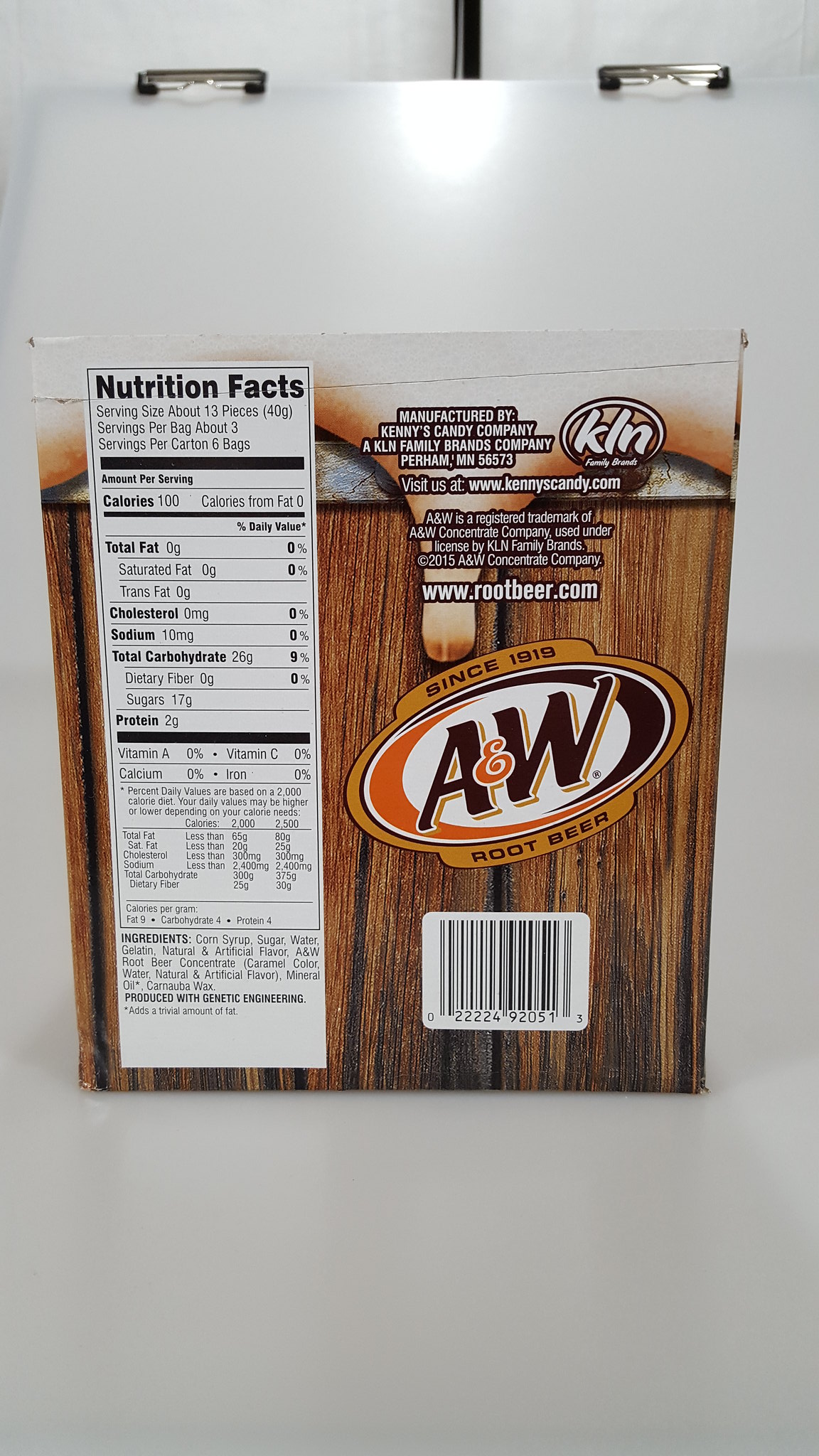This image showcases the back of an A&W Root Beer product box. The box has a wood-like brown and black design, characteristic of A&W's branding. Prominently featured is the A&W Root Beer logo in an oval shape, signaling the brand's established history with the text "Since 1910" or possibly "Since 1810." On one side of the box is a detailed nutrition facts label, which lists the serving size as 13 pieces and mentions servings per bag and bags per carton. This suggests the product might be candy or fruit snacks rather than syrup. Below the nutrition facts section, there's a list of ingredients. The right side of the image includes a circled "K-N" and further detailed branding information. At the bottom, you can see the product's barcode and its numbers. The entire image has a square aspect ratio.